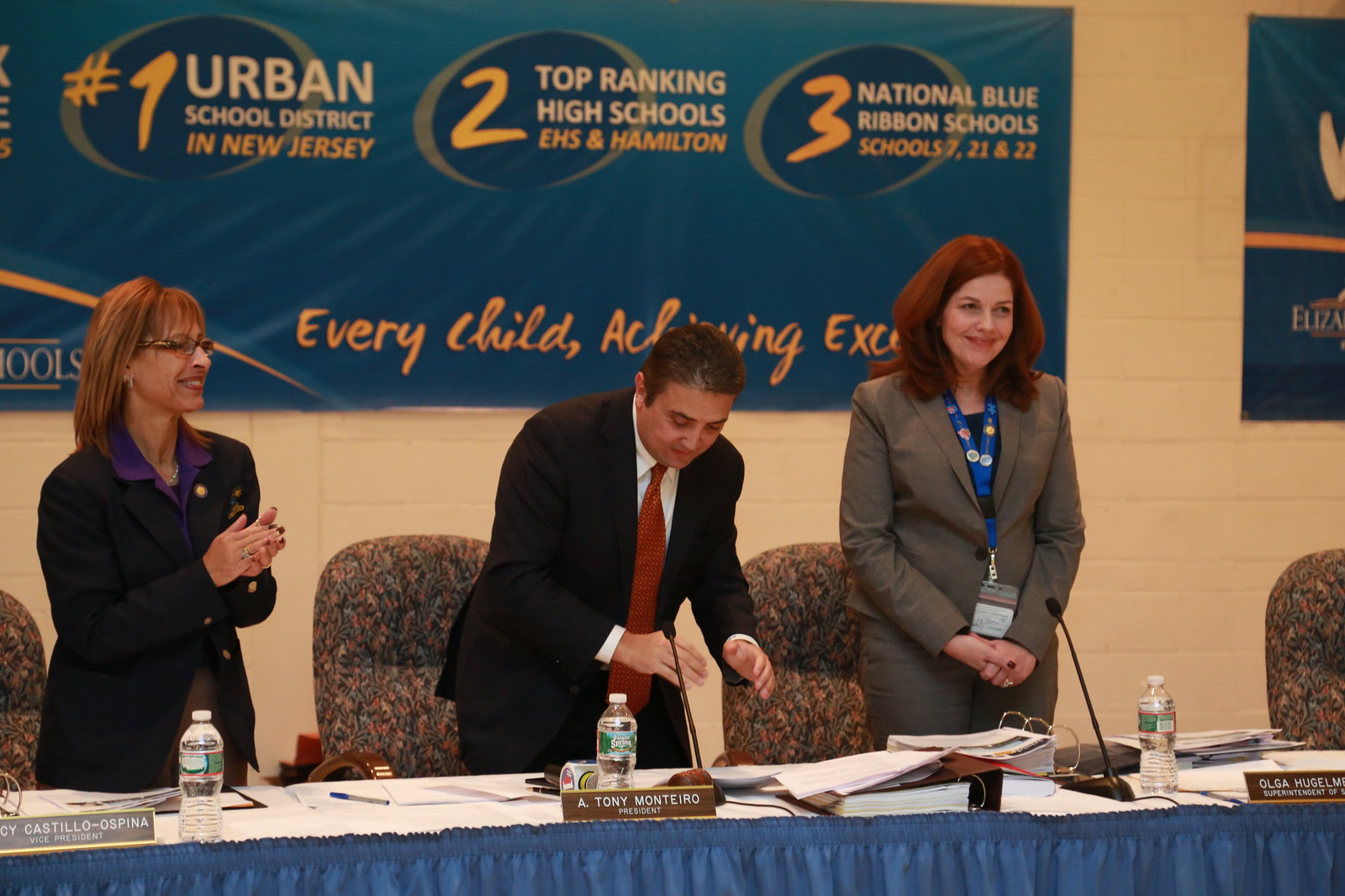This is a full-color photograph of three professionally dressed individuals, likely in their 30s or 40s, standing behind a long white table covered with a blue tablecloth at what appears to be an indoor school board meeting. The table has ring binders with numerous pages, name placards, and plastic water bottles in front of each person. Behind them, three floral print chairs are visible. The trio consists of a woman in a black suit on the left, clapping her hands; a man in a dark suit with a red tie in the middle, looking down and flipping through papers; and another woman in a gray pantsuit on the right, smiling at something off-screen. A large blue banner on the white wall behind them reads, "Number one Urban School District in New Jersey, Two Top-Ranking High Schools: EHS in Hamilton, Three National Blue Ribbon Schools: Schools 17, 21, and 22," and "Every Child Achieving Excellence." This detailed setup indicates a significant educational event celebrating achievements in the district.